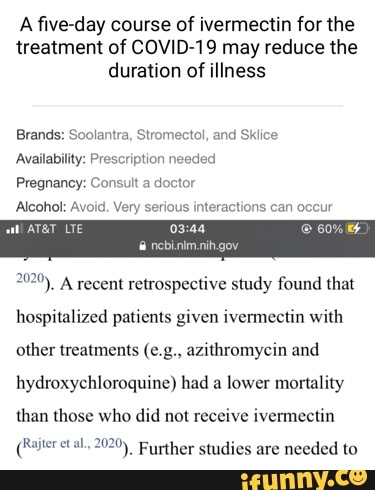In this image, the viewer is presented with a screenshot of a webpage displaying the beginning of an article titled "A five-day course of ivermectin for the treatment of COVID-19 may reduce the duration of illness." Below the title, headings such as "Brands," "Availability," "Pregnancy," and "Alcohol" are listed. The "Brands" section mentions Soolantra, Stormacol, and Skylease. The "Availability" section states that a prescription is needed. The "Pregnancy" section advises consulting a doctor, while the "Alcohol" section warns to avoid alcohol due to very serious interactions.

The background below these headings is dark gray and features typical cell phone interface icons. On the left, the signal strength is shown along with "AT&T" and "LTE." The center displays the time as 3:44, and the right corner shows a battery percentage of 60%.

The URL of the webpage is visible at the bottom of the screen. The beginning of the article mentions that a recent retrospective study found that hospitalized patients given ivermectin, along with other treatments like azithromycin and hydroxychloroquine, had a lower mortality rate compared to those who did not receive ivermectin. The text ends abruptly, suggesting further studies are needed.

At the bottom of the image, there is a black strip running from side to side. On the right side of this strip, the word "ifunny" is displayed in bright yellow text with the letter "o" depicted as a smiley face.